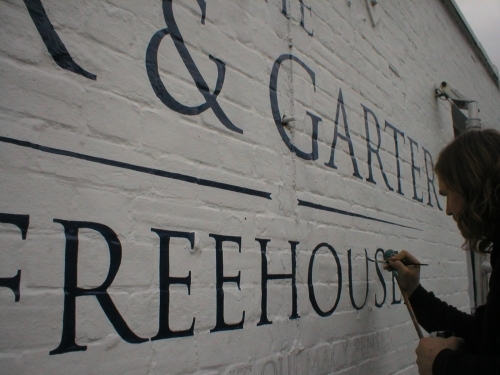The photograph depicts a scene set outdoors, featuring a white-painted brick wall adorned with blue text. The text, partially obscured, reads "Ann Garter" on the top line and "Freehouse" on the line below. A man is positioned in the bottom right corner of the image, in the act of meticulously painting the letter "U" from "Freehouse" with a thin paintbrush in his right hand, while possibly holding a paint can in his left. The paint appears darker in some areas due to the lighting. The man, with long brown hair obscuring much of his face, is dressed in a long-sleeved black shirt. Above him, there is a security camera mounted on the wall. The setting suggests the creation of a hand-painted sign or label on the exterior of a building, indicating perhaps its name or type.